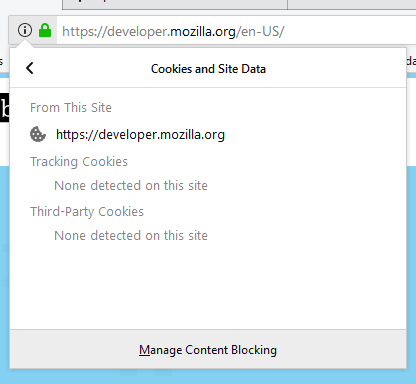The image is a zoomed-in screenshot of the URL bar from a Firefox browser, primarily focusing on the left-hand section of the bar. The URL visible is from the developer documentation site for Mozilla, specifically `developer.mozilla.org/en-US`. The URL bar itself is depicted in a sleek, chrome silver color. Key elements highlighted in the screenshot include the information (i) icon and a green lock icon, indicating that the site is secure.

Upon clicking the information icon, a drop-down menu has appeared on the screen, set against a white background. This menu provides details about the site's cookies and site data. The text within the drop-down states: "Cookies and Site Data" and specifies that no tracking cookies or third-party cookies are detected from the site `developer.mozilla.org`. This detailed security information reassures users about the safety and privacy measures of the visited site.